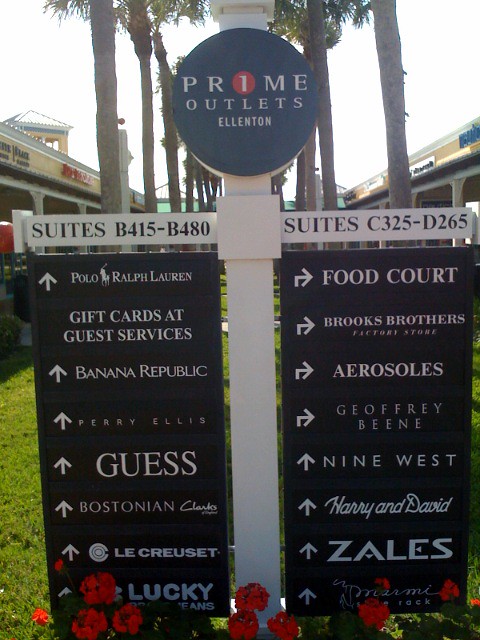The image showcases a directory sign for Prime Outlets, Ellenton, prominently featuring a blue circle with the text "Prime 1 Outlets Ellenton" with the "1" stylized in a red circle. This directory is set on a white T-post with crossbars. The left side lists suites B415 to B480, while the right side lists suites C325 to D265. Both sides have hanging blue panels denoting store information. 

The left panel directs visitors straight ahead to Polo Ralph Lauren, gift cards at guest services, Banana Republic, Perry Ellis, Guess, Bostonian, and Le Creuset. Some text is obscured by flowers but references a store with a clover icon, likely referring to Lucky Jeans.

The right panel directs visitors to the food court, Brooks Brothers, Aerosoles, Geoffrey Beene, Nine West, Harry and David, and Zales, with some text partially obscured by red flowers. The sign is framed by a well-manicured green lawn and surrounded by a covered walkway typical in outdoor shopping complexes.